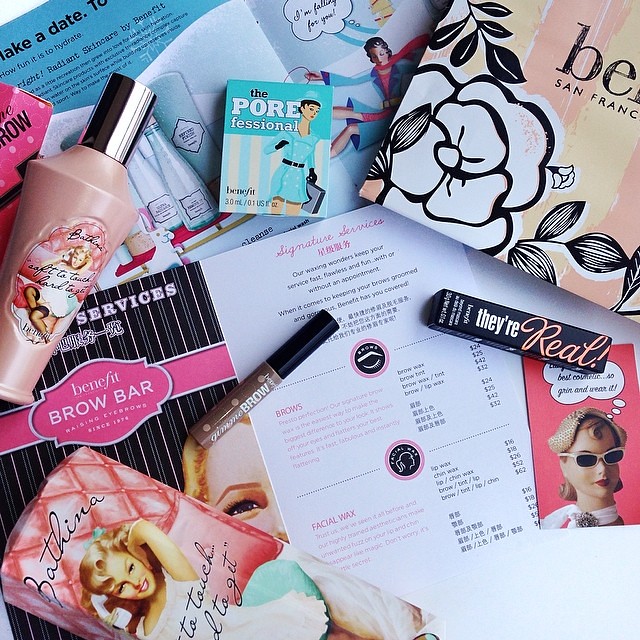The photograph features an assortment of beauty products and accompanying pamphlets arranged on a table. In the upper right-hand corner, there is a distinct pink and yellow striped box with black and white floral patterns inscribed "Benefit San Francisco." Adjacent to it lies a small blue box labeled "The Porefessional by Benefit," positioned atop an illustrated pamphlet detailing other products and their usage. Next, there is a pink bottle with a silver cap, decorated with an image of a woman and black writing. Beside it sits a pink box adorned with pink polka dots, black stripes, and black lettering. Beneath these items rests another pamphlet titled "Benefit Brow Bar," which appears to be a service menu listing various brow and facial treatments along with their prices, written in black and pink text. On top of this pamphlet is a brown tube with a black cap labeled "brow," presumably containing an eyebrow makeup product, and a black box that reads "They're Real." In the lower left-hand corner of the photo, there's a pink box featuring an illustration of a blonde woman posing with her right arm behind her head, identified by the writing "Bathina," accompanied by white cursive text. The overall arrangement is complemented by a large white sheet of paper displaying item names and prices, some listed in both English and possibly Asian text, hinting at a bilingual price guide for the services offered.